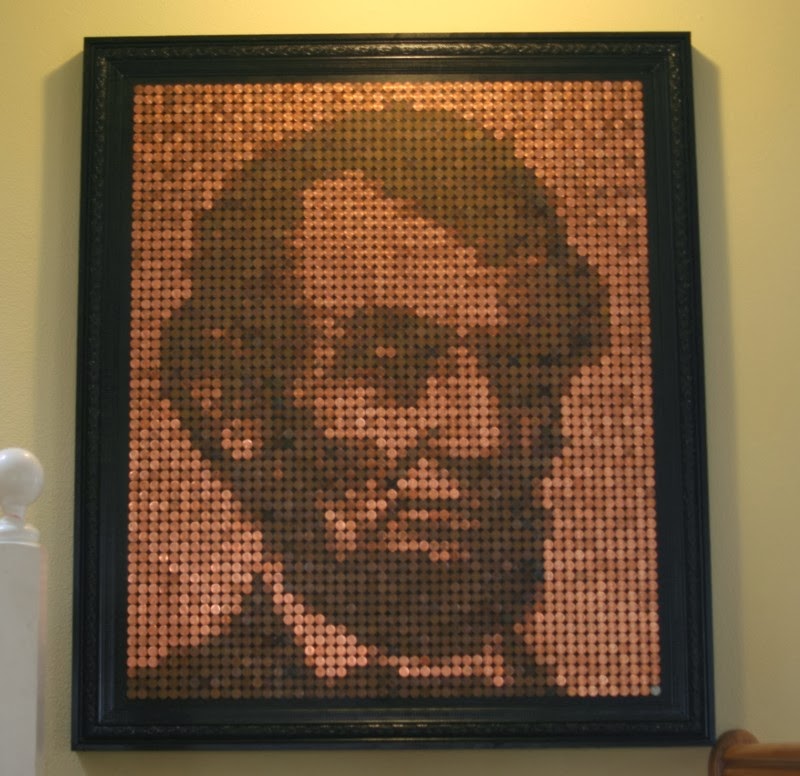This detailed photograph showcases a framed piece of artwork featuring a portrait of Abraham Lincoln. The artwork appears to be created using numerous pennies, with darker coins forming Lincoln's hair, beard, eyes, suit, and outline, and shinier coins filling in the lighter facial features and his collar. The portrait is encased in an intricately carved black wooden frame, which hangs on a softly illuminated, light yellow wall. In the top part of the image, a light source beams down, highlighting the detailed craftsmanship. On the left side of the image, there is a white bedpost with a knob at the end, while at the bottom right corner, a brown knob or railing is visible. Lincoln's expression shows him looking off into the distance, not particularly engaged with the viewer.